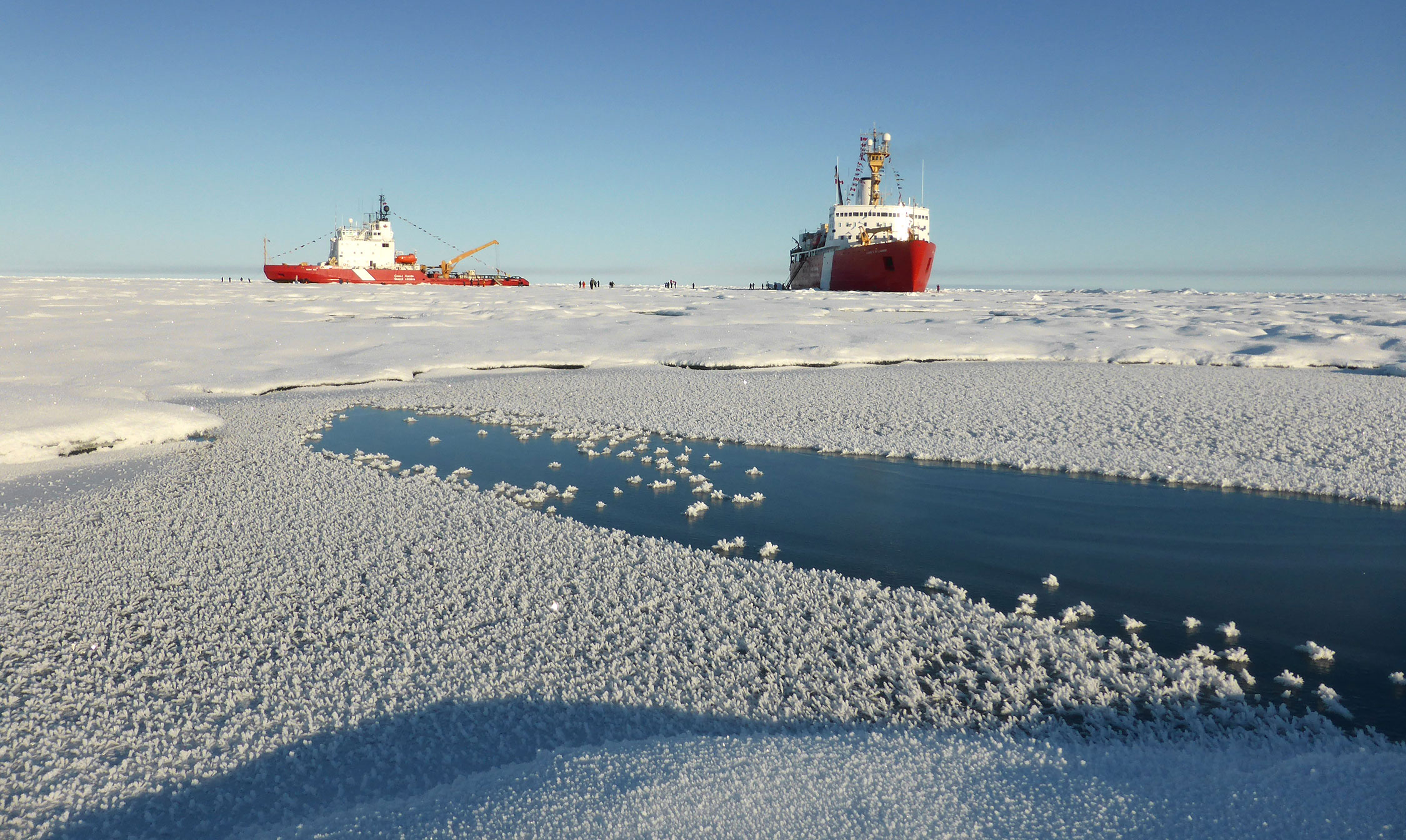This detailed outdoor photograph captures a striking scene of two large red and white ships navigating a frozen tundra where the ocean surface is predominantly covered in white snow. The left ship presents its side view, while the right ship displays its front view. Both vessels, with red bases and white upper areas, stand out against the blue water that peeks through the snow's dominion. Visible on the snow and ice surrounding the ships are individuals, possibly scientists or sailors, gathered for an indeterminate purpose. The sky overhead is a clear blue, adding to the crisp, cold ambiance of the setting. The ships appear substantial and majestic, hinting at the challenging and potentially perilous nature of navigating these icy, Arctic-like waters.